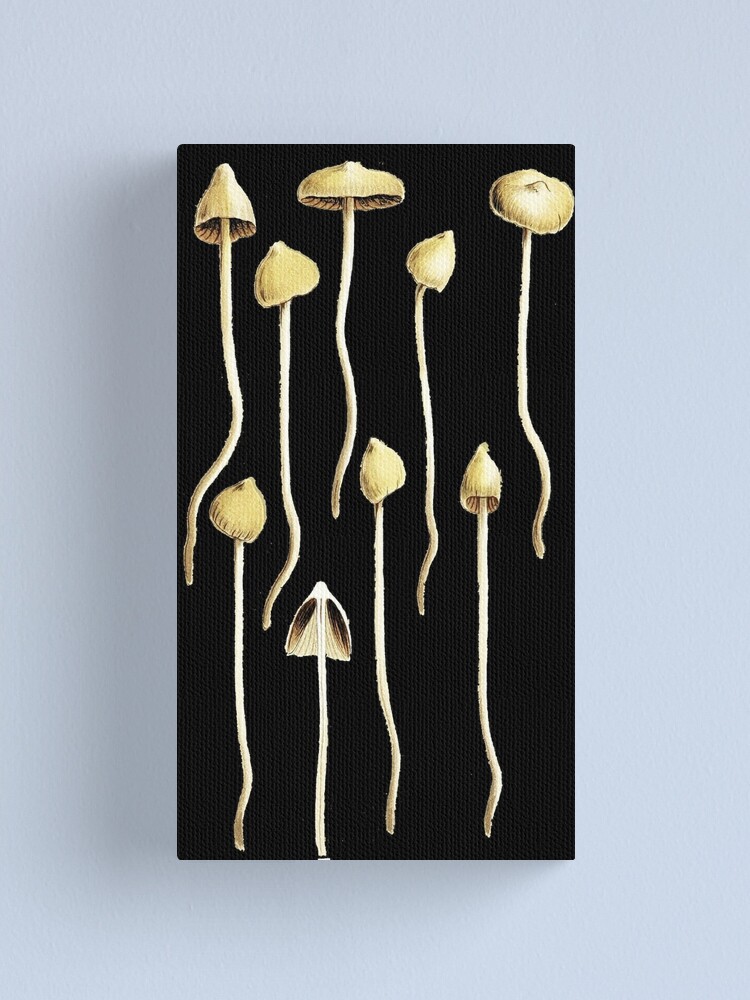This image is a detailed, meticulously painted illustration of mushrooms set against a stark black background. The painting features a total of nine mushrooms arranged in staggered lines—four along the top and four along the bottom, with an additional one in the center of the top row. The mushrooms are depicted in a light yellowish-greenish tan with long, slender stems and small, rounded caps. Notably, the second mushroom in the bottom row is uniquely illustrated with its cap partially cut away, revealing the intricate insides. The entire composition is framed within a large, gray-blue border, emphasizing the mushrooms' arrangement and adding a sense of depth to the overall depiction.